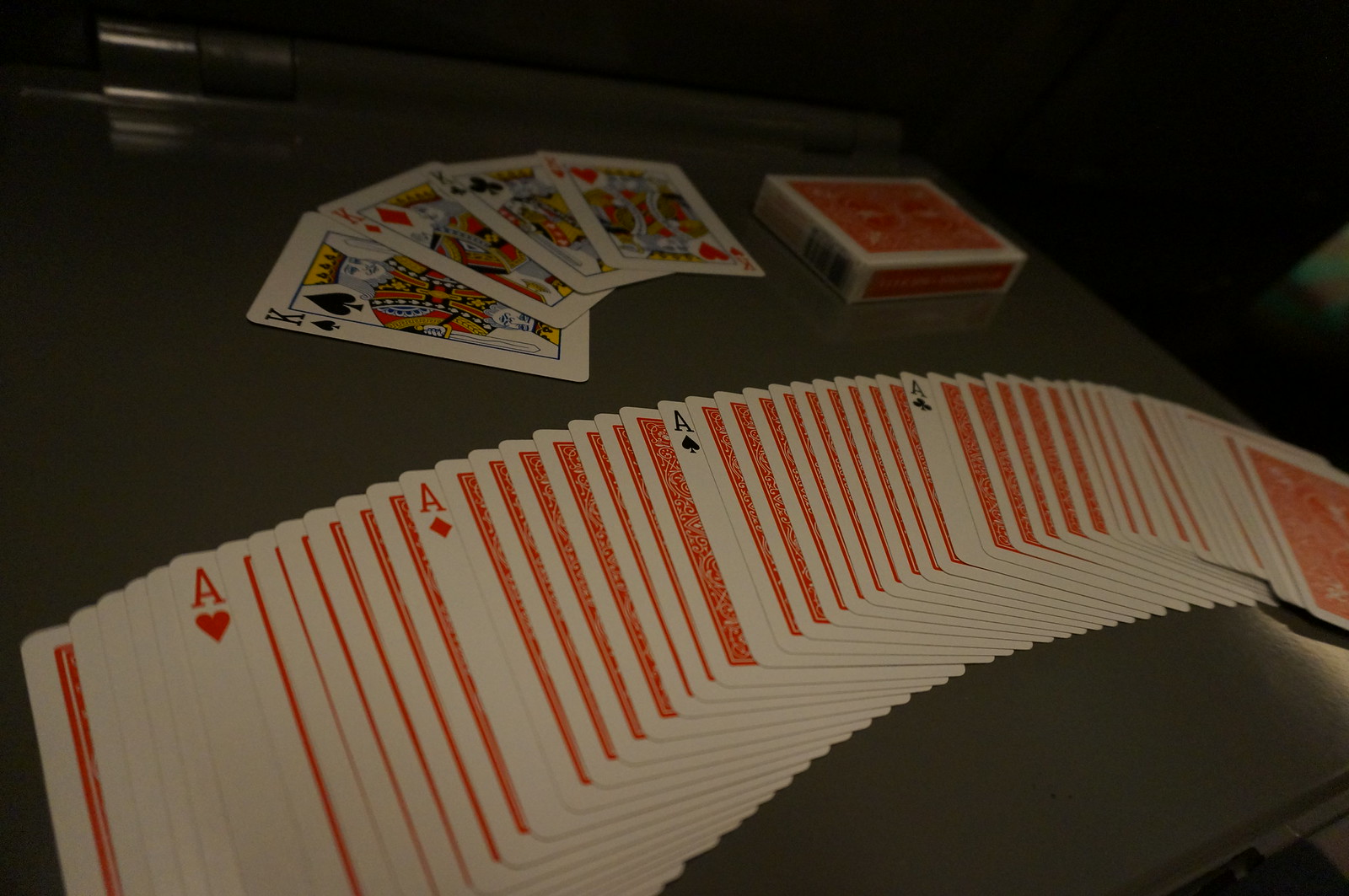The image showcases a meticulously arranged display of playing cards set against a gray tabletop. In the upper right corner, the deck's box is positioned, featuring a white backdrop with an orange cover designed to resemble the top of a playing card, prominently displaying its logo. Adjacent to the box, the four king cards - the King of Spades, King of Diamonds, King of Clubs, and King of Hearts - are elegantly fanned out. Beneath this display, the remaining deck lies face down, except for the four aces which are intentionally turned face up. From left to right, the Ace of Hearts, Ace of Diamonds, Ace of Spades, and Ace of Clubs are visible, interspersed with five or six face-down cards in between each. At the rightmost edge, a small additional stack of cards completes the arrangement, creating a visually appealing and organized scene.